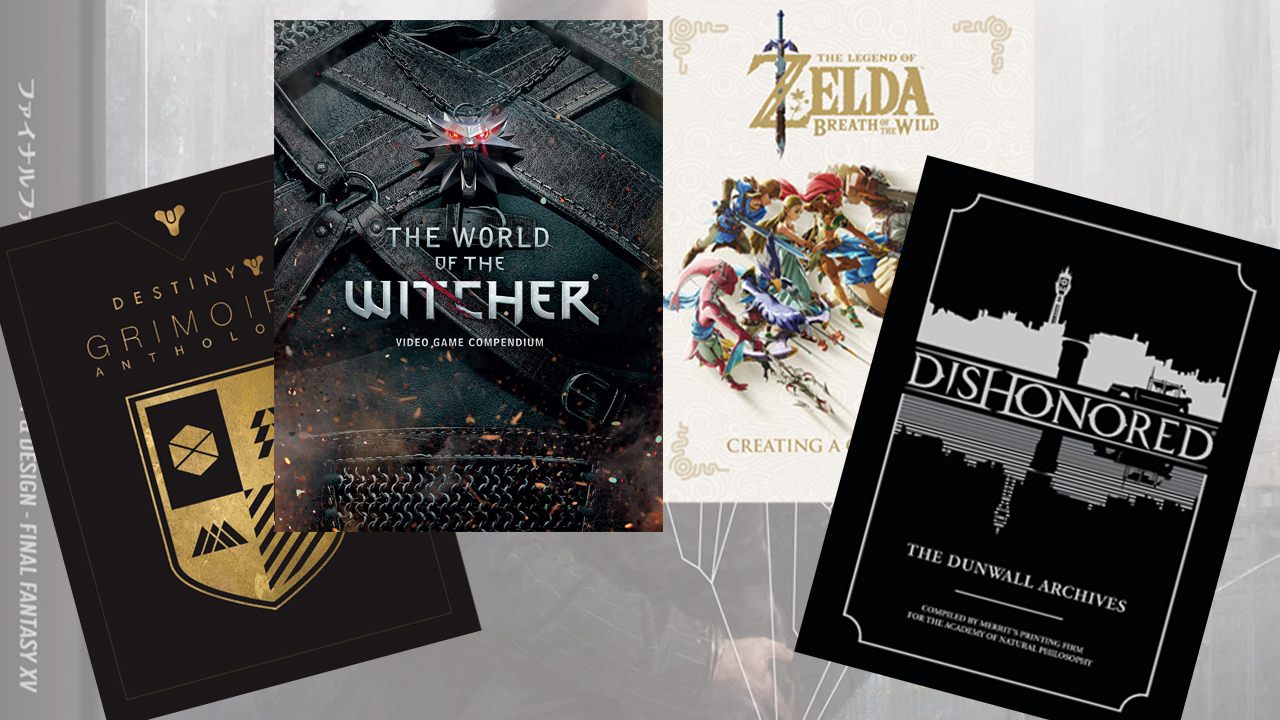The image displays four different video game books arranged from left to right. The first book, titled "Destiny Grimoire Anthology," features a black cover with gold elements, including stylized text and a golden shield logo. The second book, "The World of the Witcher Video Game Compendium," has a dark gray and black cover with a detailed background depicting leather straps and a prominent silver necklace with a growling wolf pendant that has striking red eyes. The third book, "The Legend of Zelda: Breath of the Wild," presents a cream-colored cover with gold fonts and showcases multiple brightly colored characters in a watercolor style. The last book on the right, titled "Dishonored: The Dunwall Archives," has a black cover with white text and a design that includes a black and white cutout of a cityscape reflecting a castle.